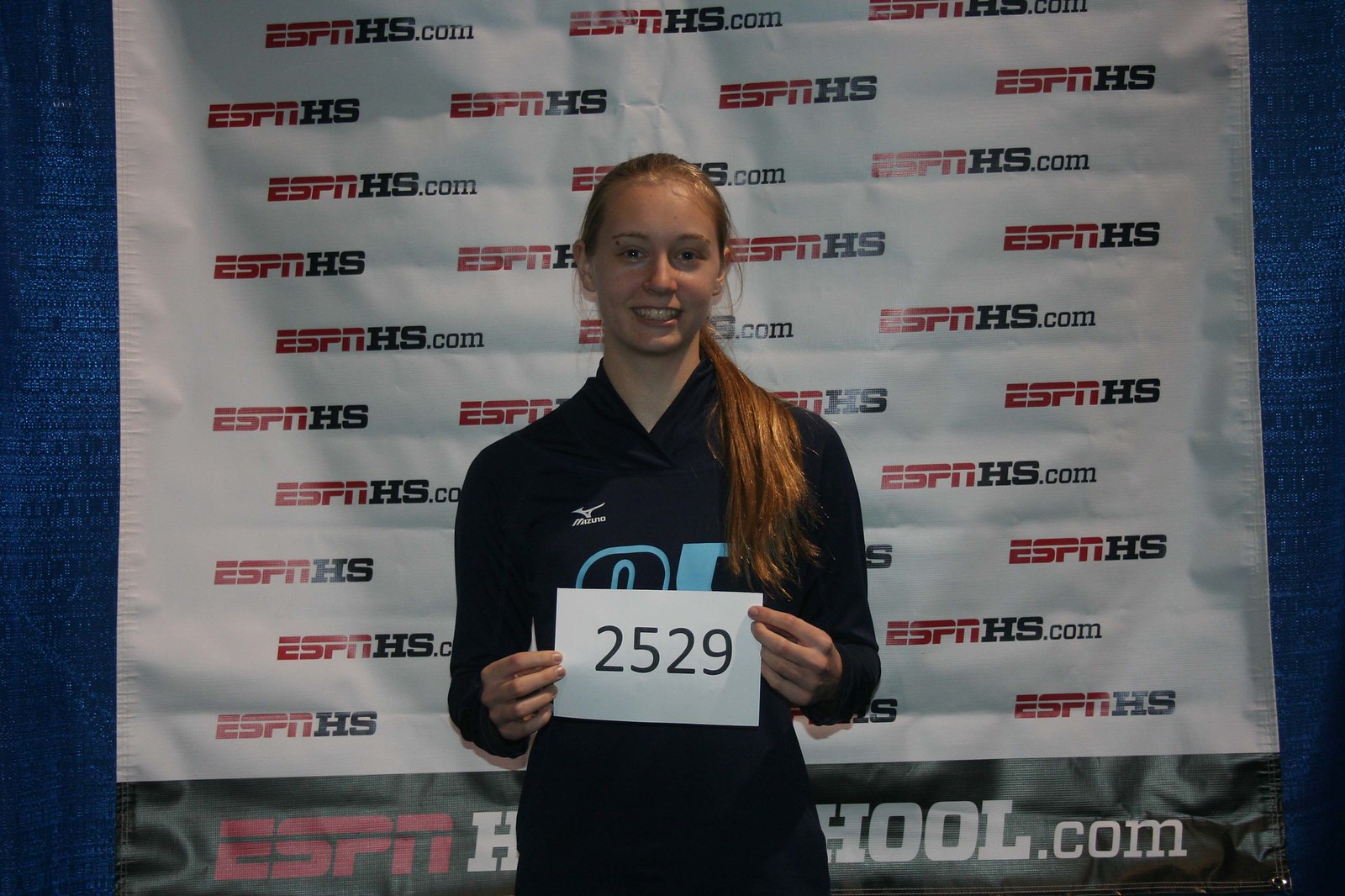The photograph features a cheerful, young Caucasian woman with orange-blonde hair tied up in a ponytail that spills over her left shoulder. She is smiling and holding a sign with the number 2529. She wears a dark, black sweatsuit with a v-neck and some unreadable text. Behind her is a large, white banner with repeating text that reads "ESPNHS" and "ESPNHS.com," in black and red lettering. This horizontal banner is plastered across a blue backdrop, creating a clear contrast with the main colors visible in the image being black, red, white, and blue.